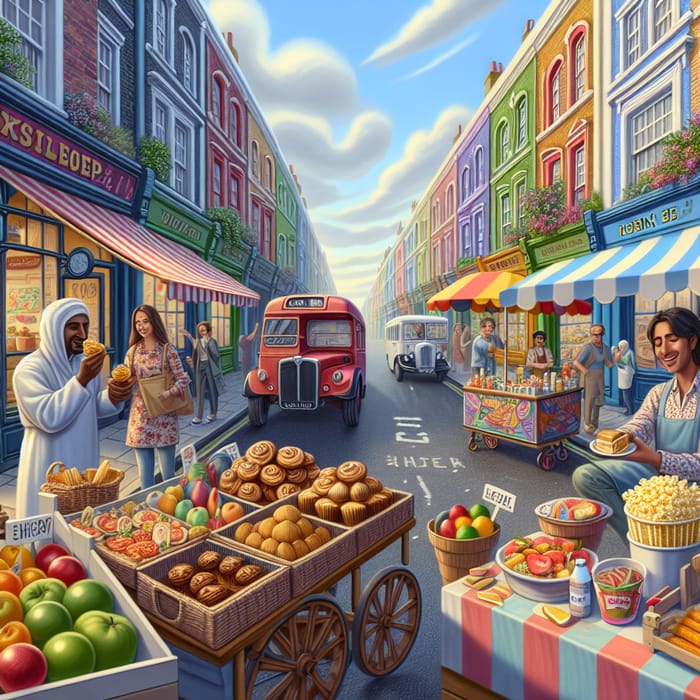This image is a colorful, animated drawing or painting of a bustling, sunny city street scene, slightly taller than it is wide. It features vibrant buildings in shades of blue, orange, green, purple, red, and white, with storefronts adorned with bright, striped awnings. The sky is a cheerful blue with fluffy white clouds.

In the foreground, various street vendors are selling an assortment of items. On the left side, a vendor in a white robe stands behind a cart brimming with baked goods and fruits like apples and oranges. A Middle Eastern man is sampling bread from this stand, while a woman in a flowered shirt and a large shoulder bag stands nearby, with another woman just behind her. Toward the right, under a striped red and blue tablecloth, another vendor offers popcorn and possibly other baked goods, alongside a cart that appears to sell drinks or ice cream.

In the background, a black street hosts a vibrant red bus followed by a white bus. The scene is lively with the presence of distorted faces among the pedestrians, adding a unique, whimsical touch to the artwork. This charming market scene captures the essence of a colorful, everyday outing in a vibrant urban setting.